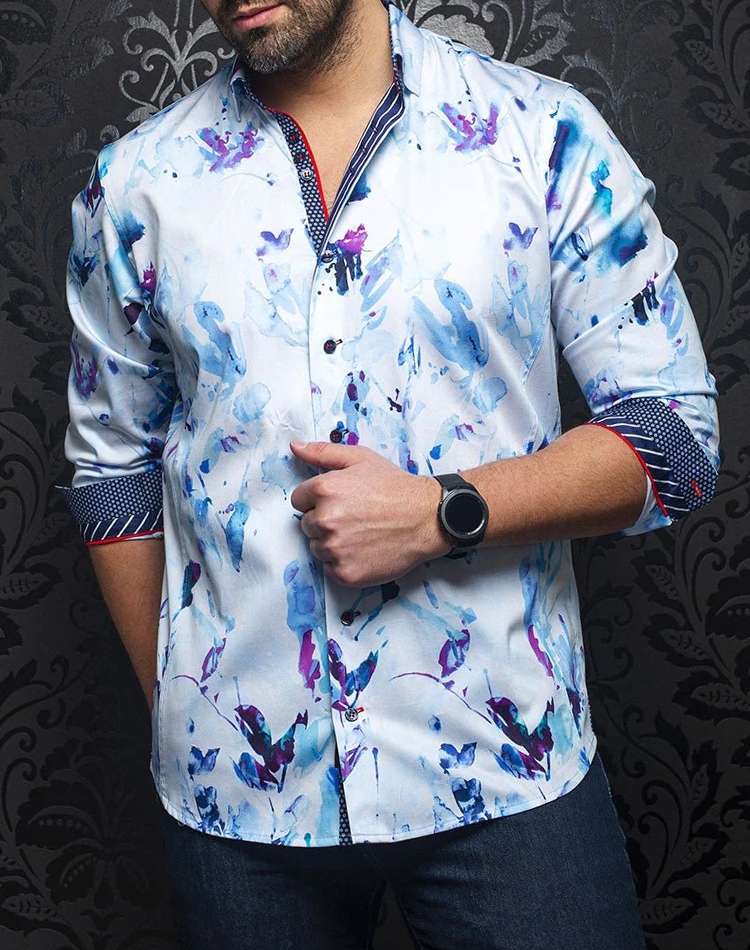The photograph features a male model posing against a matte black backdrop with glossy black filigree or floral patterns. The image is cropped just above his mouth, revealing his well-trimmed beard. He is dressed in a long-sleeve, button-down shirt that is predominantly white with intricate splashes of blue and purple, resembling watercolor or floral patterns. The button lining is adorned with dark blue and white polka dots on one side and dark blue and white stripes on the other, with similar patterns on the inside of the rolled-up sleeves. The model is wearing dark blue jeans and a black smartwatch on his left wrist, which he holds in front of his chest in a fist. The photograph captures the model standing confidently, showcasing both the detailed shirt and the sleek smartwatch.